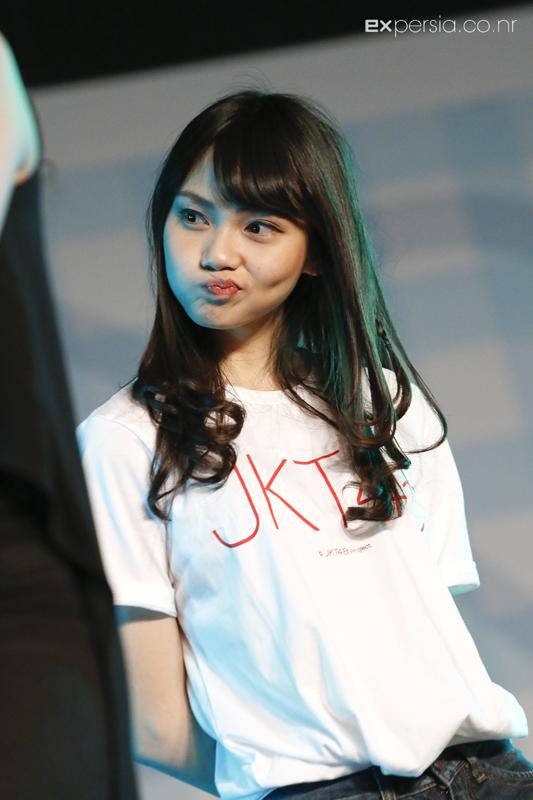The photograph features a young Asian woman in her 20s, positioned centrally and wearing a white t-shirt partially obscured by her long black hair. The visible part of the red text on her shirt reads "JKT4." She is also dressed in jeans, the top of which is just visible at the lower edge of the image. The woman's lips are pursed as if she has just tasted something sour, and she appears to be looking off to the left despite facing forward to the right. The background is blurred, adding a sense of depth, and in the top right corner, there is a watermark that reads "EXPERSIA.CO.NR." Additionally, there is a blurred figure to the left side, suggesting a busy or public setting, possibly a conference or event. The overall color palette of the image includes shades of dark brown, red, white, black, and dark blue.